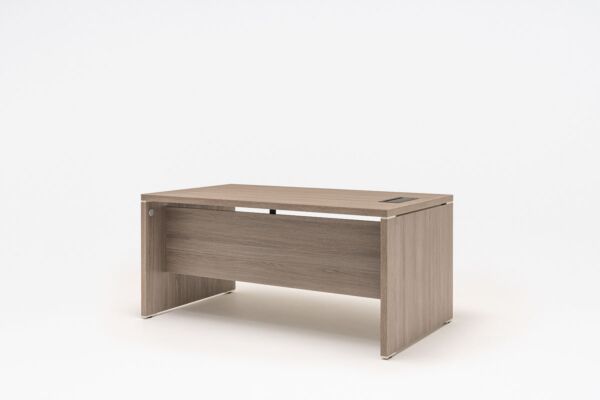The image depicts a minimalistic and simplistic wooden desk set against a plain white backdrop. The desk features a light brown, manufactured wood appearance, lacking the sturdiness of traditional hardwood furniture. It consists of a flat rectangular wooden top, supported by two side panels of the same material and color. A single horizontal wooden panel connects the two side panels at the back for added stability. This design does not include drawers, and the top right corner features a small gray indentation, though it's not deep enough to serve as a drawer. The desk's shadow is cast on the white ground beneath it, suggesting overhead lighting. The desk is the sole object in the image, devoid of any accompanying furniture or decorative elements.